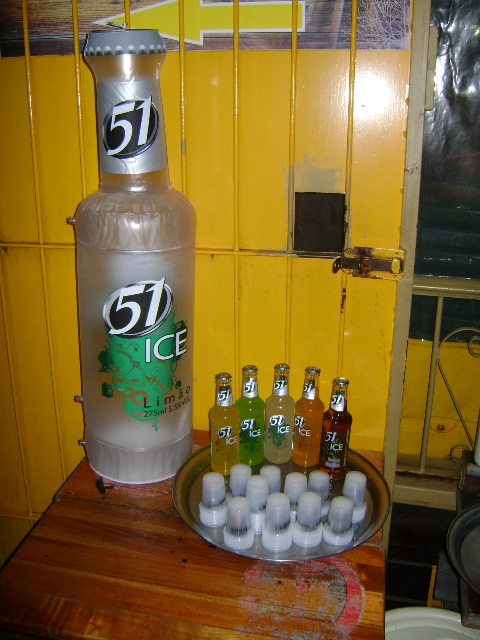The photograph depicts a brown wooden table against a yellow wall, partially framed by an open metal door with a left-facing yellow arrow with a white outline. Dominating the scene is an oversized, slightly frosty, transparent bottle labeled '51 Ice,' which might be a decorative lamp due to its size. Positioned on the left side of the table, the large bottle is accompanied by a round silver tray. This tray holds five smaller clear bottles of the same '51 Ice' brand, each containing different colored liquids: green, clearish yellow, orange, red, and another variation of orange. Also on the tray are numerous small clear glasses stacked, resembling shot glasses.